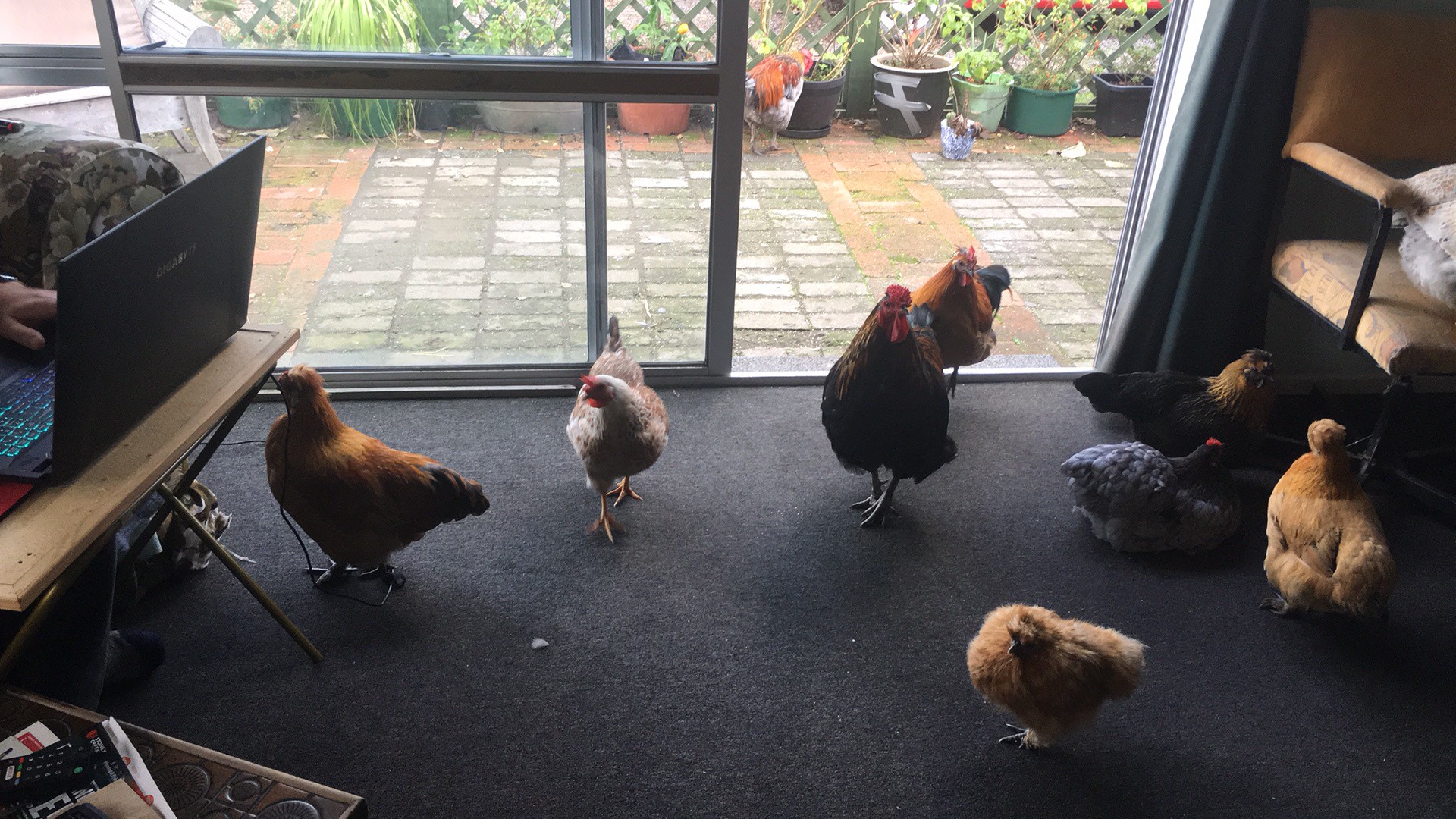The image shows a curious scene of eight chickens, along with a large rooster, inside a house. The birds are wandering on a carpeted floor, with a sliding glass door left open behind them. This door leads to a brick patio outside, adorned with potted plants against a wooden lattice fence, where a couple more chickens are seen running around. Inside the home, to the left, a person is casually working on a laptop at a table, unperturbed by the poultry guests. The house interior is dimly lit, relying on the natural daylight streaming through the open door. Nearby, there is a table cluttered with a remote and a pile of magazines. The chickens inside are of various colors, including white, brown, and reddish-orange, with a few baby chicks among them.